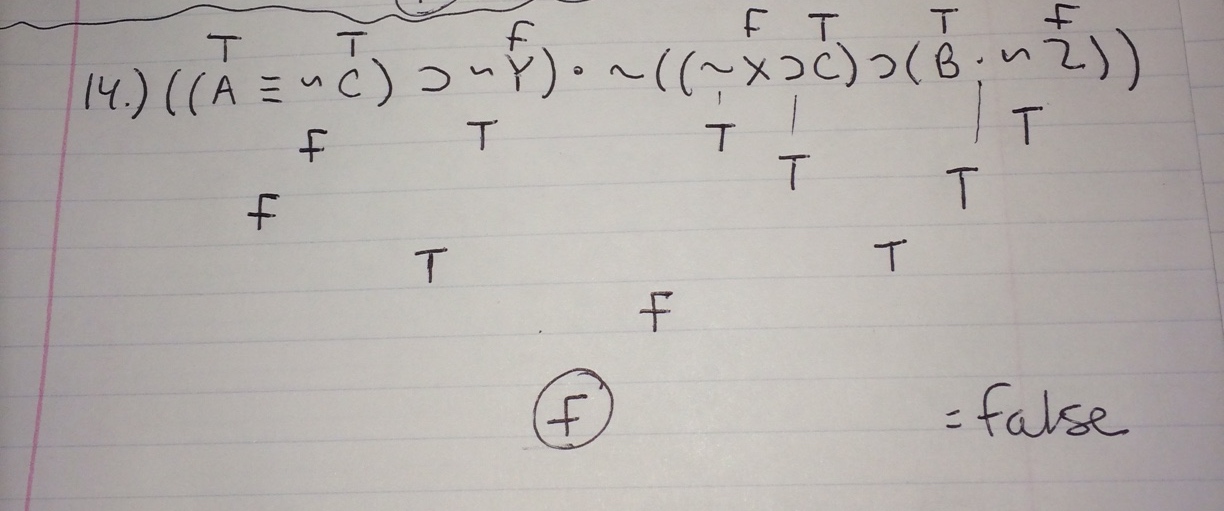The image depicts a close-up view of a white sheet of ruled paper, reminiscent of an exercise book, featuring light blue horizontal lines. Meticulously written on the paper is a complex set theory equation that interweaves a variety of letters and mathematical symbols. The equation is as follows: 

\[ 14 \left( \left( A ≡ C \right) ∩ Y \cdot \left( \left( X ∩ C \right) ∩ B ≡ Z \right) \right). \]

This notation suggests a detailed exploration into set theory, which is a branch of mathematical logic that deals with sets, or collections of objects. The equation encapsulates interactions and relationships between multiple variables, indicated by the symbols for equivalence (≡), intersection (∩), and others, reflecting a high level of mathematical sophistication.